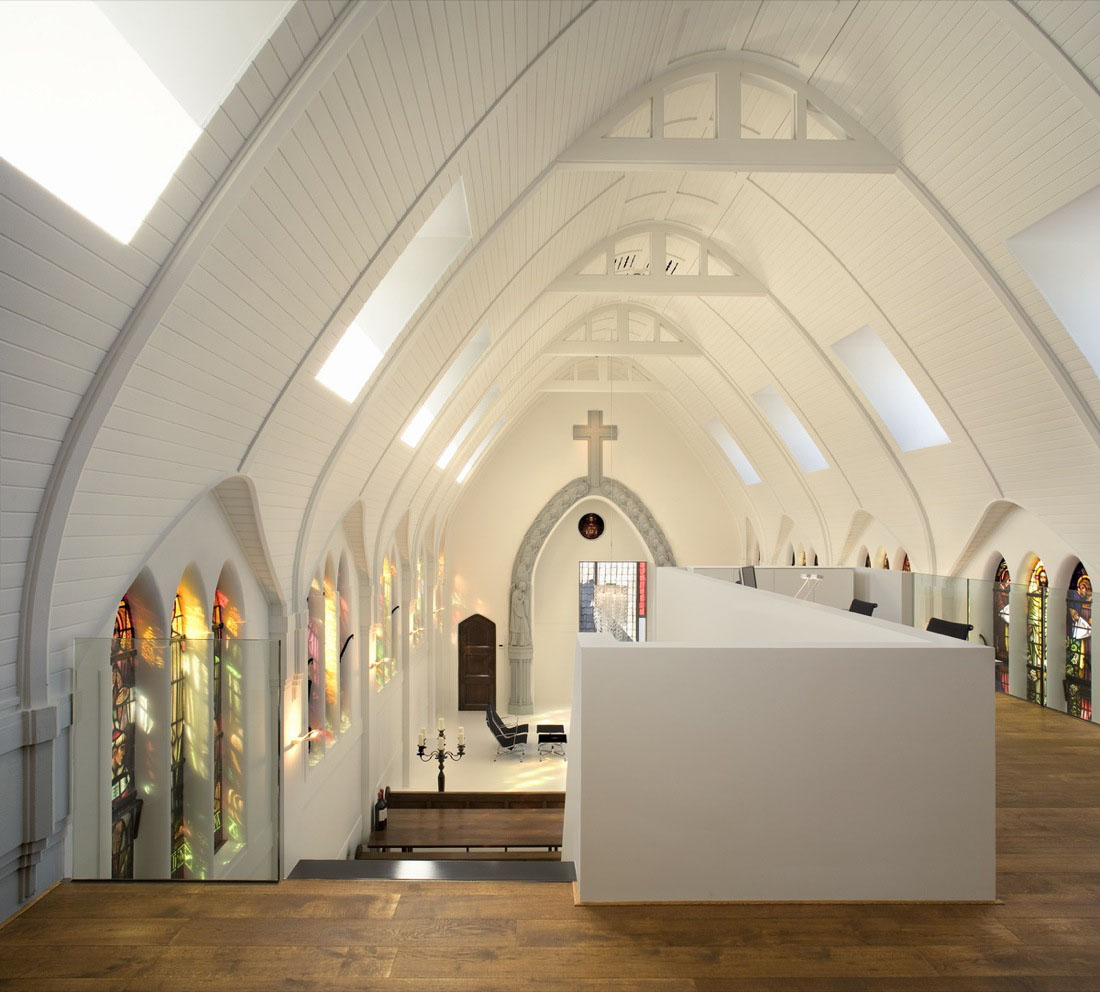This is a color photograph of the interior of a modern, spacious church, viewed from an elevated balcony area above the sanctuary. The ceiling is notably high and features white, vaulted arches with skylights that permit ample natural light. The church's walls are predominantly white, adding to the sense of space and purity. 

On both sides of the church are sets of tall stained glass windows which display an array of colors including pink, yellow, green, red, and orange. These colorful windows scatter vibrant light across the church's interior, creating an almost ethereal effect. Below the balcony, on the first level, there are dark wood pews, a cross over a gray archway at the front, and a small dark brown wooden door tucked to the left side. The floor is dark wood, contrasting elegantly with the lighter elements of the decor.

Obstructing part of the view from the balcony is an L-shaped white wall, which blocks some of the pulpit and podium area. To the right, another white wall hides part of the seating area, yet some dark chairs and a glass railing are still visible. This glass railing overlooks the stained glass windows on the right side, while on the left, the stained glass windows are clearly visible and vividly catch the sunlight. 

Additionally, we can see hints of church furnishings such as two small tables, several chairs potentially for the choir or other uses, and a large iron candelabra positioned near the front of the sanctuary. The ceiling also has some ventilation features. The overall impression is one of serene beauty and modern elegance within a traditional church setting.